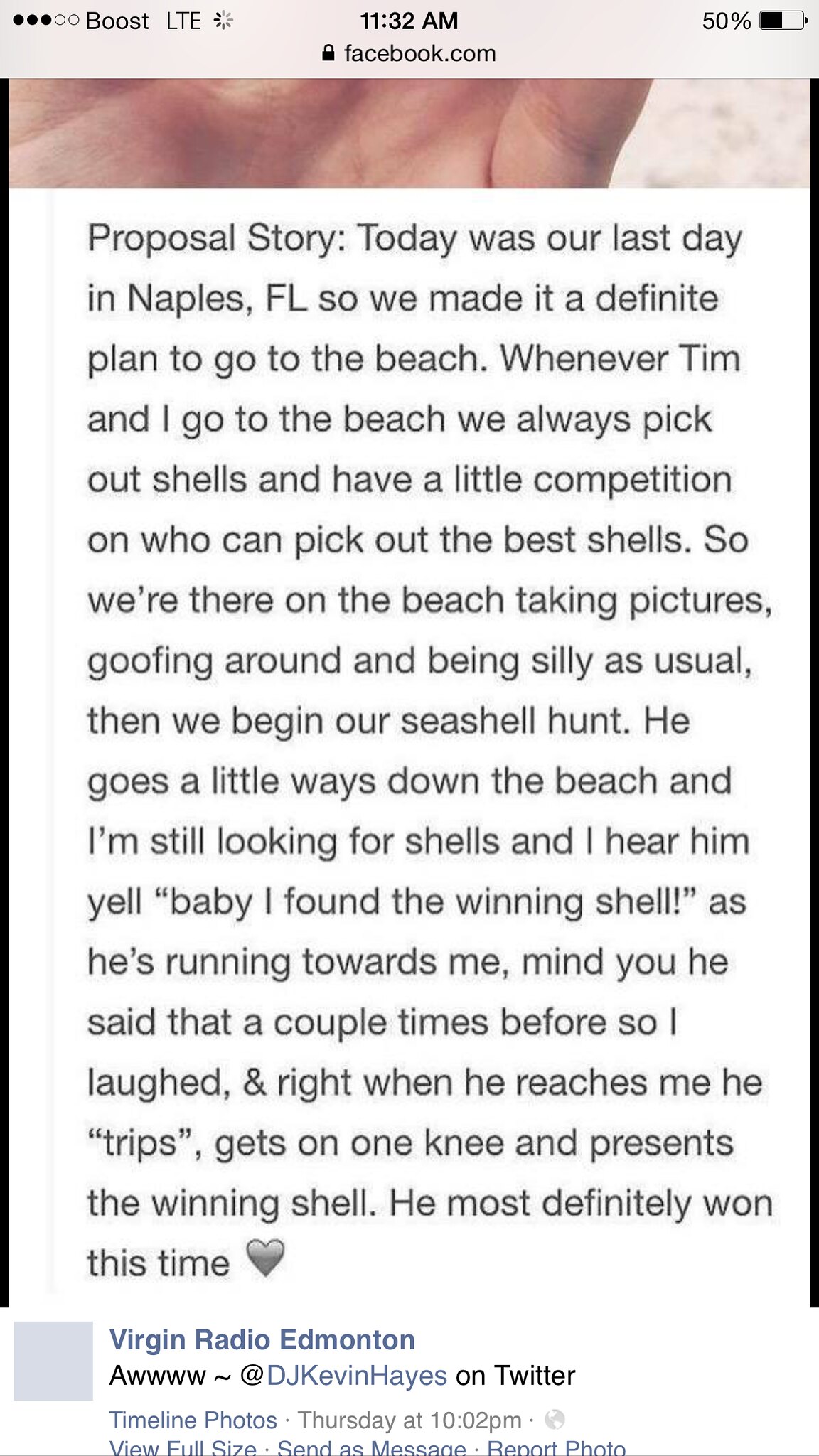A detailed caption for the image combining and refining the three provided descriptions might be:

"The image shows a screenshot taken from a smartphone at 11:32 AM on facebook.com, with 50% battery life and Boost LTE as the service provider. At the top of the screen, part of a human hand is visible, and there is a paragraph with a white background and black text titled 'Proposal Story.' The text narrates a memorable day in Naples, Florida, where a couple, Tim and the narrator, spent their last day at the beach. They indulged in their usual fun, taking pictures, being silly, and engaging in a competitive seashell hunt. Tim, having wandered a bit down the beach, shouts that he found the winning shell and runs towards the narrator. Despite having joked about finding the best shell before, this time his enthusiasm is different. He trips, gets on one knee, and presents a shell, marking his proposal. The story concludes with the note that Tim 'most definitely won this time,' punctuated by a grey, heart-shaped emoji. Additionally, the post includes a reference from Virgin Radio Edmonton, with DJ Kevin Haynes expressing delight over the heartwarming story on Twitter."